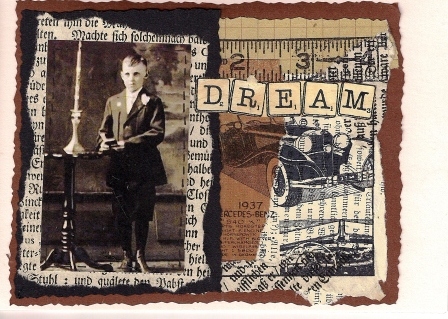The image is a meticulously crafted collage, predominantly in black and white with sepia tones, set in a landscape orientation. It features two main portrait-oriented images. On the left, there's an old, grainy, black and white photograph of a young boy from what appears to be the 19th century, dressed in a formal suit, short socks, shoes, and a boutonniere, standing next to a table with a lit candle. This is layered over torn paper edges with a mix of brown and black colors, and above it is text resembling old English calligraphy from newspaper prints. On the right side of the collage, there's a black and white line drawing of an antique car, pointed towards the right, underlined by an image of part of a ruler. Above the car are beige squares spelling out the word "DREAM" using Scrabble-like tiles. The background of the entire collage is a dynamic mix of torn and pasted brown and black papers, along with various pieces of newsprint, contributing to a vintage, handcrafted aesthetic.